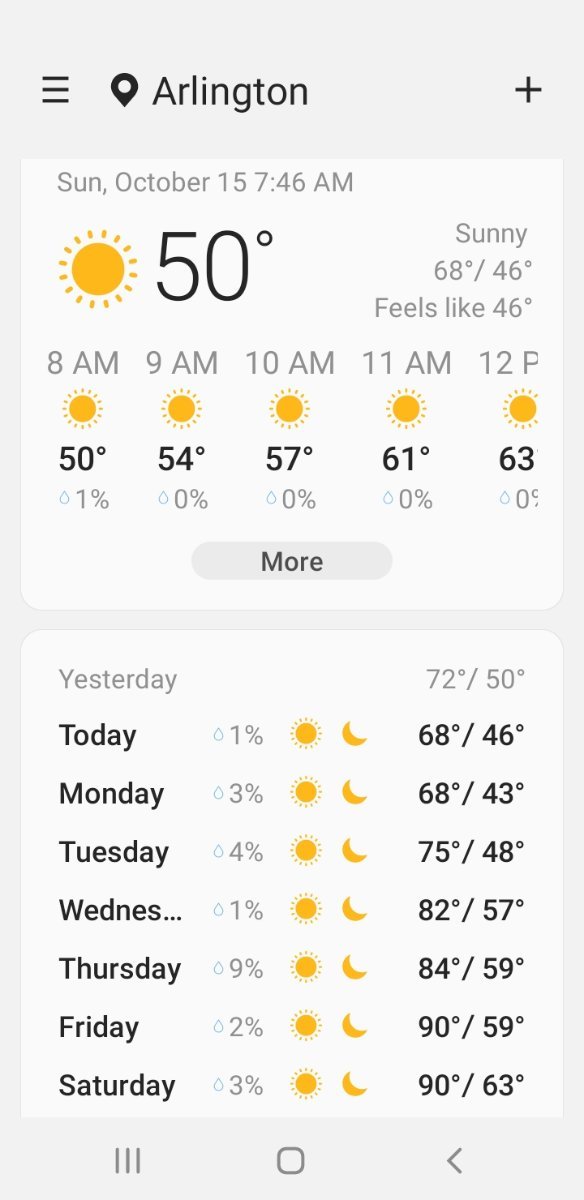The image features a weather forecast interface set against a gray background. In the top left corner, there is a hamburger menu icon, followed by a location pin indicating Arlington. On the right side of the screen, there is a plus symbol. 

Below this, a white square displays the date and time, reading "Sunday, October 15, 7:46 a.m." Next to this, a sunny icon is shown with the current temperature of 50°F. The weather summary notes a sunny day, with a high of 68°F and a low of 46°F, and indicates that it "feels like" 46°F.

Below the summary, an hourly forecast lists temperatures and precipitation chances: 
- 8 a.m.: 50°F, 1% chance of precipitation
- 9 a.m.: 54°F, 0% chance of precipitation
- 10 a.m.: 57°F, 0% chance of precipitation
- 11 a.m.: 61°F, 0% chance of precipitation
- 12 p.m.: 63°F, 0% chance of precipitation

A button labeled "More" is located beneath this hourly forecast.

Further down, another section provides a brief outlook with three days:
- Yesterday: High of 72°F, low of 50°F
- Today: High of 68°F, low of 46°F
- Monday: High of 68°F, low of 43°F
- Tuesday: High of 75°F, low of 48°F